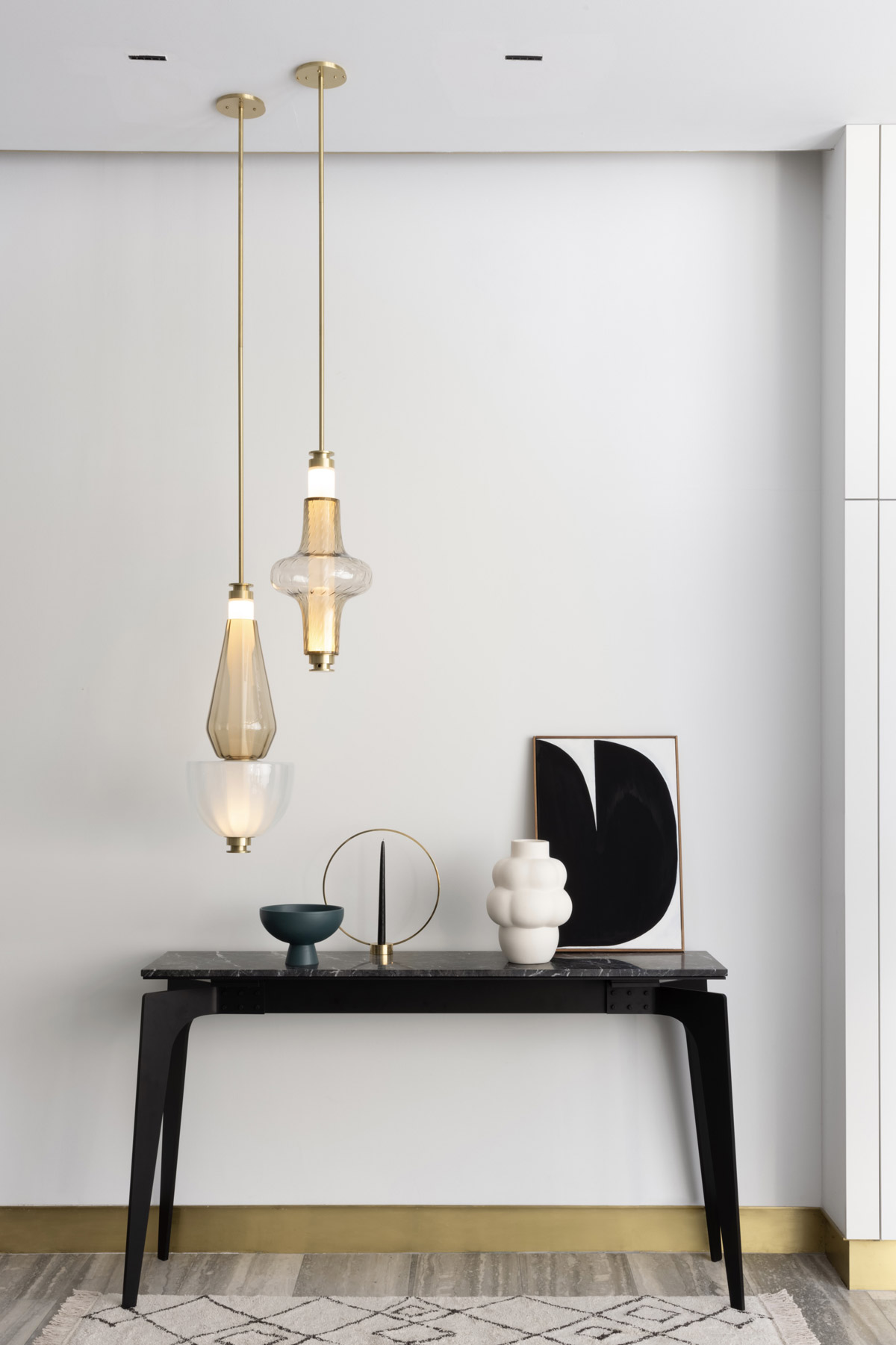The image captures a detailed interior scene focused on the lower portion of a room featuring a gray hardwood floor embellished with a white rug adorned with black diamond patterns. Against a white wall with a golden baseboard, there is a narrow black table supported by angled black legs and topped with a black marbled surface. Placed on the table are various objects including a unique black dish with an inverted cone base, a sculptural gold circle with a black cone centerpiece, and a distinctive white vase with rounded ball shapes around its base transitioning into a white cylindrical form at the top. Additionally, a piece of geometric artwork framed in gold, consisting of two sideways half-moon black shapes, adds an artistic touch. Above the table, two hanging light fixtures descend from the white ceiling, each suspended by golden tubes attached to golden discs. The left lamp features a dark frosted glass cover emitting an orange glow, combined with an upside-down white frosted glass dome glowing at the bottom. The right lamp, positioned slightly higher, displays a white frosted glass bulb tapering to a cone at both ends, also casting an orange light.